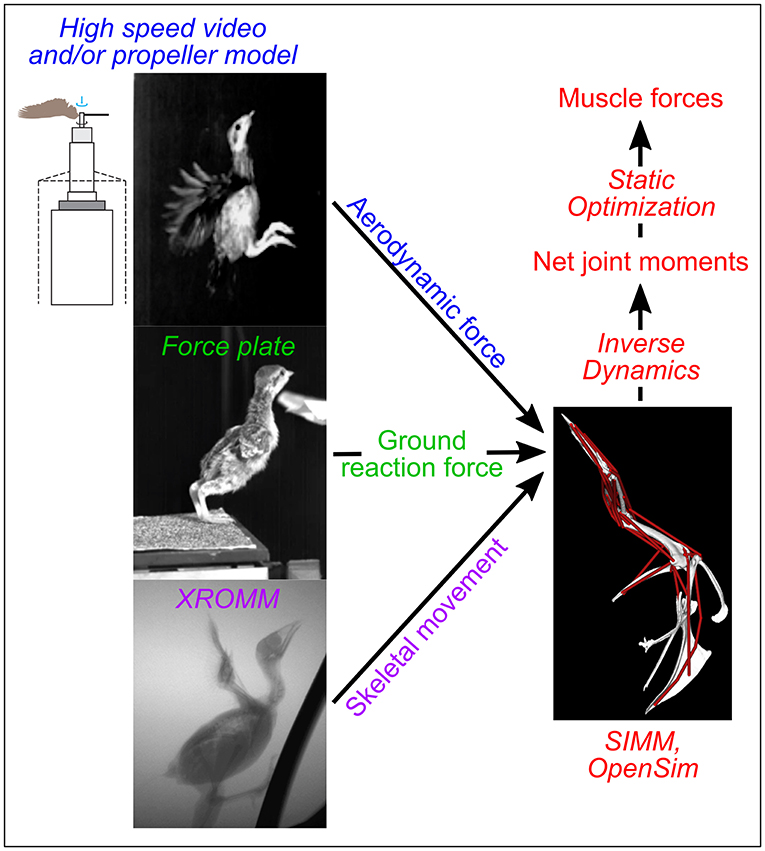This scientific infographic, reminiscent of a textbook illustration, features both photographs and diagrams on a clean white background. In the top left, a photograph shows a bird (likely a young chicken or fledgling) jumping into the air, set against a black background with blue text reading "high-speed video and/or propeller model." Below, another photograph labeled "force plate" depicts the bird standing with its neck extended and wings outstretched, possibly trying to fly. The bottom left contains an X-ray image tagged "XROMM," capturing the bird's skeletal structure with its wings spread.

Black arrows extend from these three photographs, annotated with "aerodynamic force," "ground reaction force," and "skeletal movement," all pointing towards the right side of the infographic. Here, a schematic diagram featuring a line drawing of the bird's skeleton, outlined in red, is labeled with advanced biomechanical terms such as "SIMM, Open SIMM," "inverse dynamics," "net joint movements," "static optimization," and "muscle forces." These elements collectively illustrate the biomechanical forces and skeletal movements involved in the bird's flight mechanics.